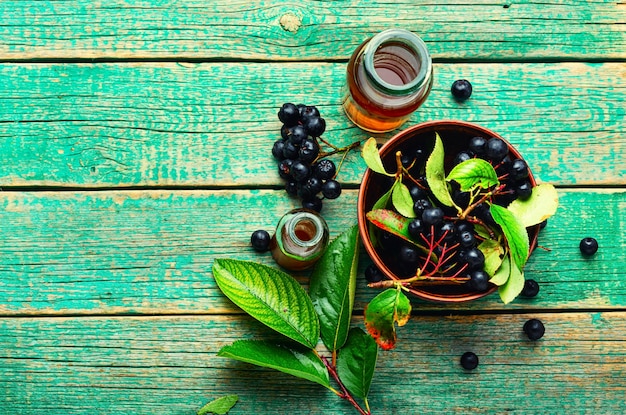This photograph, taken from a top-down perspective, captures an array of objects meticulously arranged on a weathered wooden table, painted with a faded green hue that allows the natural wood color to peek through. At the heart of the image is a large, circular bowl with a copper-toned rim, containing a branch adorned with glossy green leaves and clusters of almost black berries, interspersed with dark pink-red stems. Surrounding the bowl, various other elements are artfully placed: to the top left, a cylindrical glass jar filled with an amber-hued liquid, likely honey, and to the left, a smaller jar also containing the same golden fluid. Scattered around are additional berries, some attached to stems and others lying loose on the table. At the bottom center of the photo, another stem lies with a cluster of these nearly black berries, accompanied by a few vibrant green leaves.